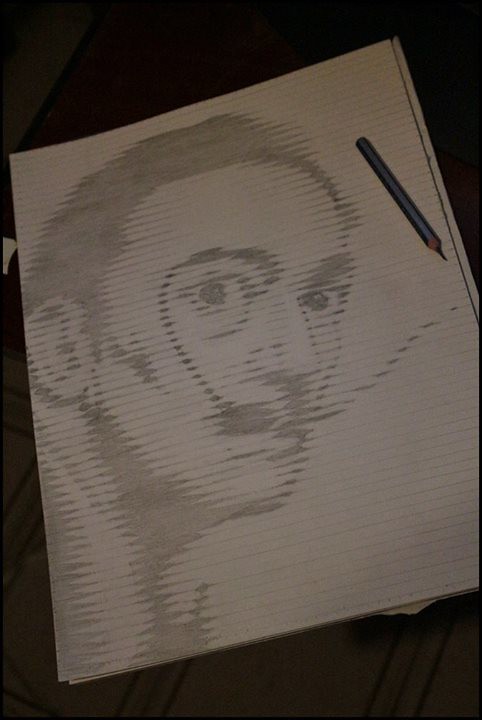This image showcases an open sketchbook lying on a tiled floor. The floor features predominantly white tiles with a reddish tile accentuated by a black border at the top. Natural lighting illuminates the scene, casting a dramatic ambiance without the use of artificial lighting. The sketchbook contains parallel horizontal lined paper, which is slightly folded at one end. Resting atop the pages is a small blue pencil with an exceptionally sharp tip. The sketch on display is a meticulously drawn portrait of the renowned Spanish artist Salvador Dalí, complete with his iconic mustache. The portrait, rendered in gray tones, exhibits a slightly blurred, almost ethereal quality. Dalí’s visage is turned to the right, but his wide, piercing eyes gaze directly at the viewer, complemented by his dark, distinctive hair.